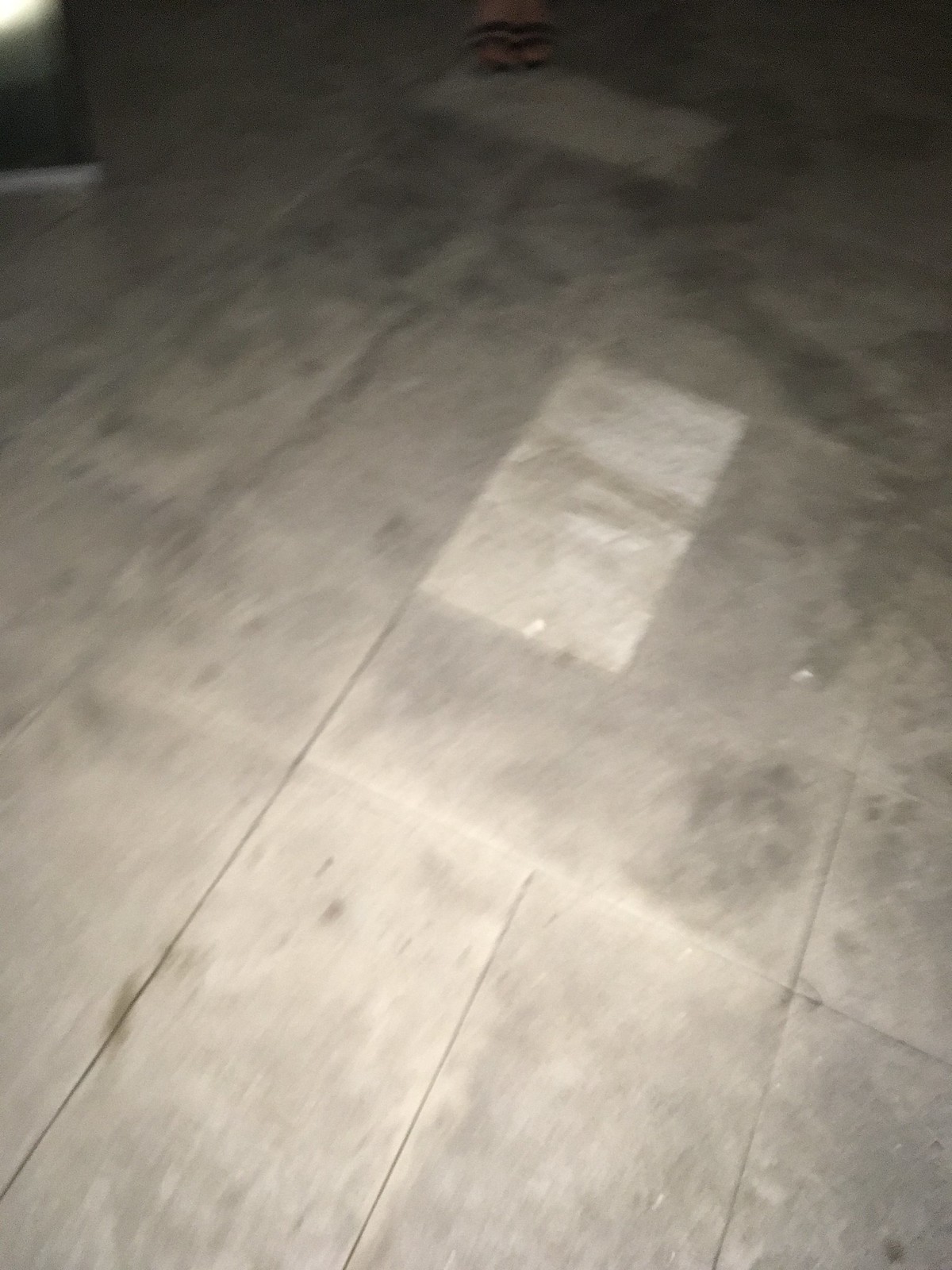The photograph captures an out-of-focus and dimly lit scene of what appears to be a patio floor composed of rectangular pavers. The pavers are set closely together, touching but not mortared, suggesting a laid, rather than tiled, construction. The foreground pavers appear gray, fading to black towards the upper portion of the image, indicating a dark area illuminated by a flash that only reaches the foreground. In the center of the image, there is one notably brighter paver amidst the surrounding ones. Similarly, at the very top center, another paver stands out as significantly brighter compared to its adjacent counterparts, despite the overall dark tone of that area.